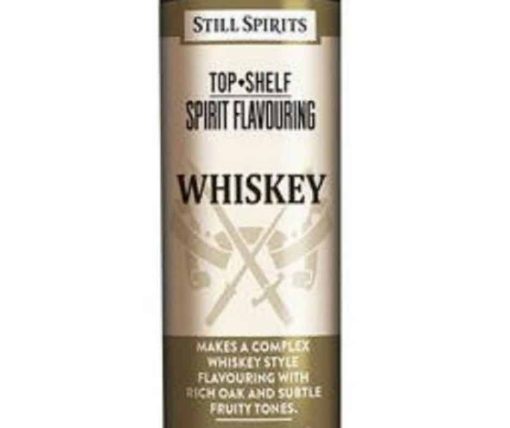This detailed label for a bottle of whiskey by Still Spirits, prominently features the brand name "Still Spirits" at the top, followed by "Top Shelf Spirit Flavoring." The central part of the label displays the bold word "Whiskey" with a coat of arms design beneath it, including two crossed swords. The label's color scheme primarily consists of gold, beige, black, and white. Gold bars frame the top and bottom of the label, while the middle section has a light beige background. At the very bottom, a description states, "Makes a complex whiskey style flavoring with rich oak and subtle fruity tones." The design and colors suggest a luxurious and refined product likely displayed in a liquor store.